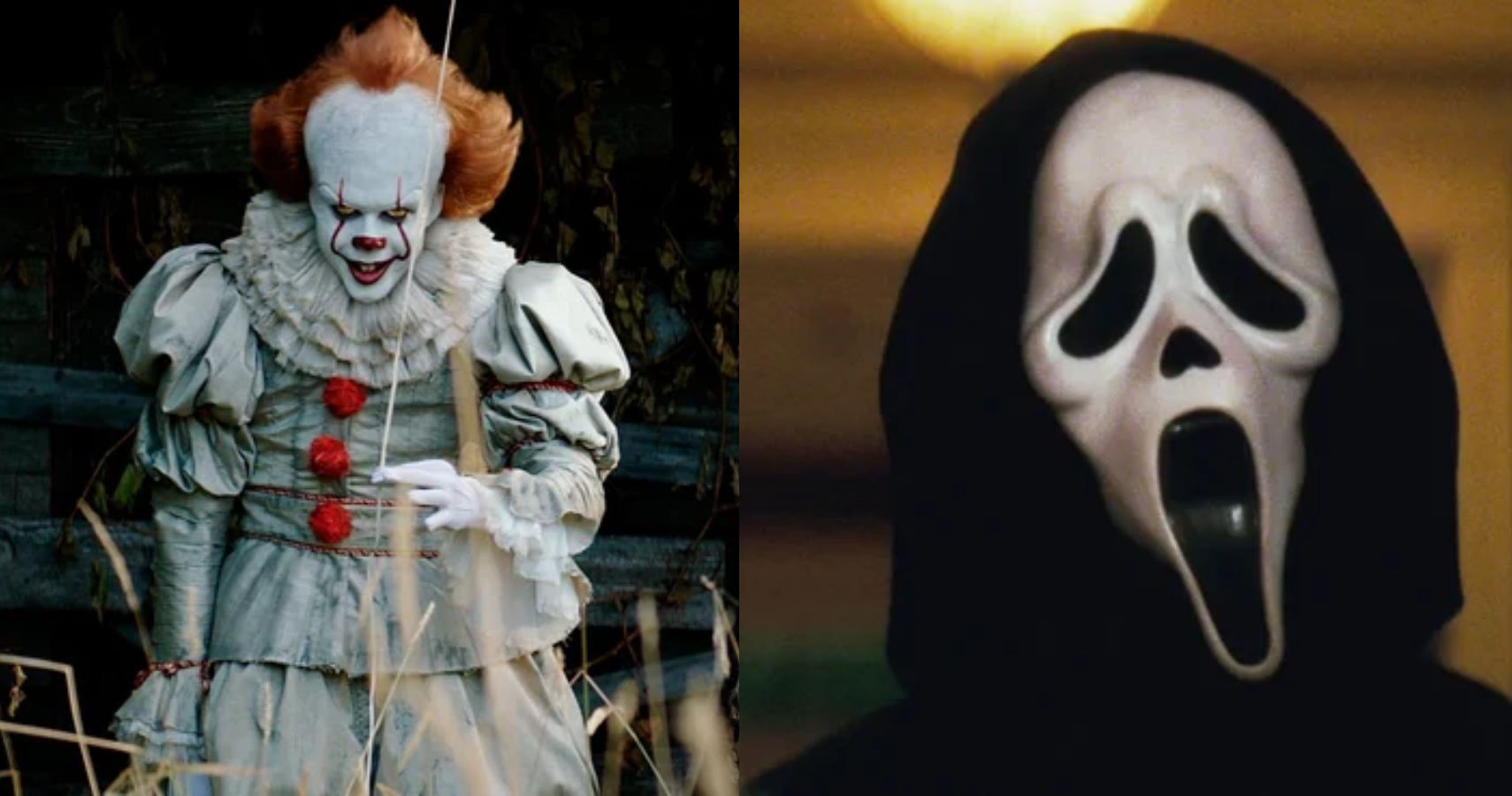The image is a professionally shot, full-color composite comprising two separate indoor scenes lit with artificial lighting, each depicting iconic horror movie characters. On the left side is the modern version of Pennywise from the Stephen King movie "IT" (2020s adaptation). Pennywise, with his white face paint and red lipstick, is instantly recognizable by his wild red hair. He dons an old-fashioned, bluish-white clown costume adorned with white ruffles and red pompom buttons, complemented by a ribbed waist and baggy pants. Despite his traditionally playful attire, his menacing eyes and the streaks of red paint trailing from his eyes to his mouth add to his terrifying demeanor. On the right side stands Ghostface, the eerie antagonist from the "Scream" franchise. This figure is cloaked in a black hooded outfit, with a haunting white mask resembling a misshapen Grim Reaper's face. The mask features exaggerated black eye holes and a gaping mouth, evoking a perpetual scream. This juxtaposition of horror icons creates a chilling Halloween-themed visual.